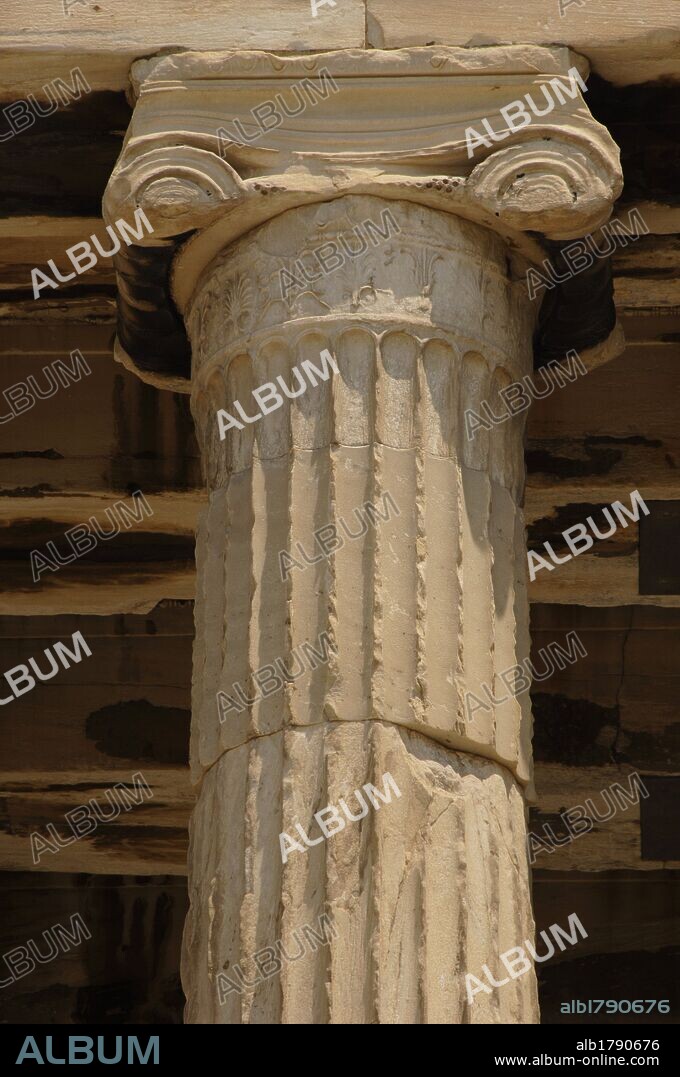The image is a detailed close-up of the top of a column, likely from an old coliseum or building. The column's material appears to be a light tan stone or white marble, with vertical ribbing running up and down its surface. The top of the column is adorned with ornate scrolls at each corner, resembling carved "cinnamon roll" shapes in clay or stone.

There is notable damage to the column, with some chunks missing, and it is made up of multiple sections stacked atop one another. The background features a brownish hue with horizontal lines that vary in white, green, and tan shades.

Prominently displayed across the image is a white, diagonal watermark that reads "ALBUM" in all capital letters. In the bottom left corner, a long black rectangle contains the text "ALBUM" in light blue. To the right within this rectangle, there are additional inscriptions: "ALB1 790676" and "www.album-online.com." The overall composition is marked by contrasting shadows cast by the column's ridges and the intricate background.